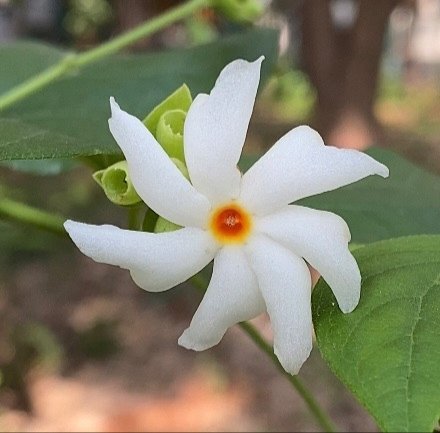In this slightly granular and pixelated square color photograph, we are presented with a delicate white flower dominating the center of the frame, its seven waxy petals spiraling like pinwheel blades in a clockwise direction. Each petal is an ivory white, and they radiate from a vibrant center where a deep orange merges into a yellow ring, highlighting the flower's stamen and stigma. The image, although soft in detail, captures the surrounding green foliage clearly, with heart-shaped and spear-shaped leaves in varying shades of green—darker ones in the backdrop and lighter ones to the left. Behind the white flower, the background blurs into large shapes of lighter browns and tans at the bottom, hinting at dirt and possibly tree trunks to the right, suggesting the flower's natural woodland or forest environment. To the bottom right, a mostly full green leaf is visible, while the rest of the background remains out of focus, with patches of pink and darker browns indicating the presence of more distant elements. Overall, the photograph beautifully contrasts the vibrant, detailed flower with its softer, more indistinct surroundings.